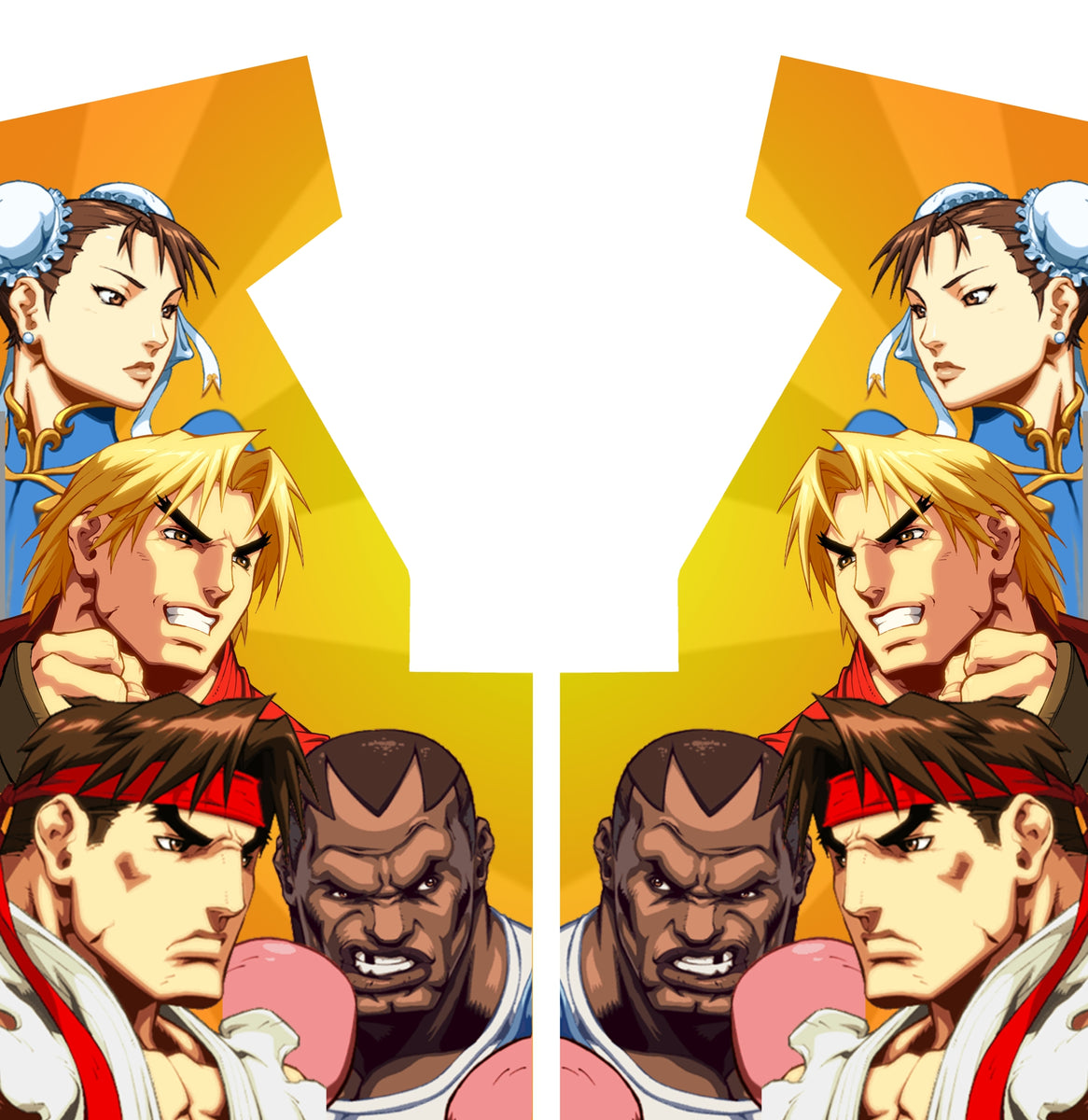This animated drawing, with bright and vibrant colors, depicts characters from the Street Fighter video game series. The image is styled to mimic the shape of an arcade console, featuring two mirror-image sides. Dominated by a yellow background, the composition includes four distinct human characters with exaggerated features, arranged to face their mirrored counterparts.

On the left side from top to bottom:
1. Chun-Li, an Asian woman with dark brown hair styled in two pigtail buns, wears a bonnet, blue high-collared top, and a pearl earring.
2. Ken, a fierce-looking man with long blonde hair and very dark eyebrows, reveals his teeth in a snarl.
3. Ryu, a man with dark hair tied back with a red bandana, wears a white karate gi and has light skin.
4. Balrog, an imposing black man with a close-cropped haircut, sporting a white shirt and baring his teeth, with one prominently missing.

Mirroring this arrangement on the right side:
1. Chun-Li appears again with her distinct attire and features.
2. Ken mirrors his fierce expression and hairstyle.
3. Ryu stands opposite with his red bandana and white gi.
4. Balrog faces inward with his recognizable missing tooth and fierce expression.

The detailed and symmetrical composition highlights the iconic characters, emphasizing their unique and defining traits within the arcade-style framework.